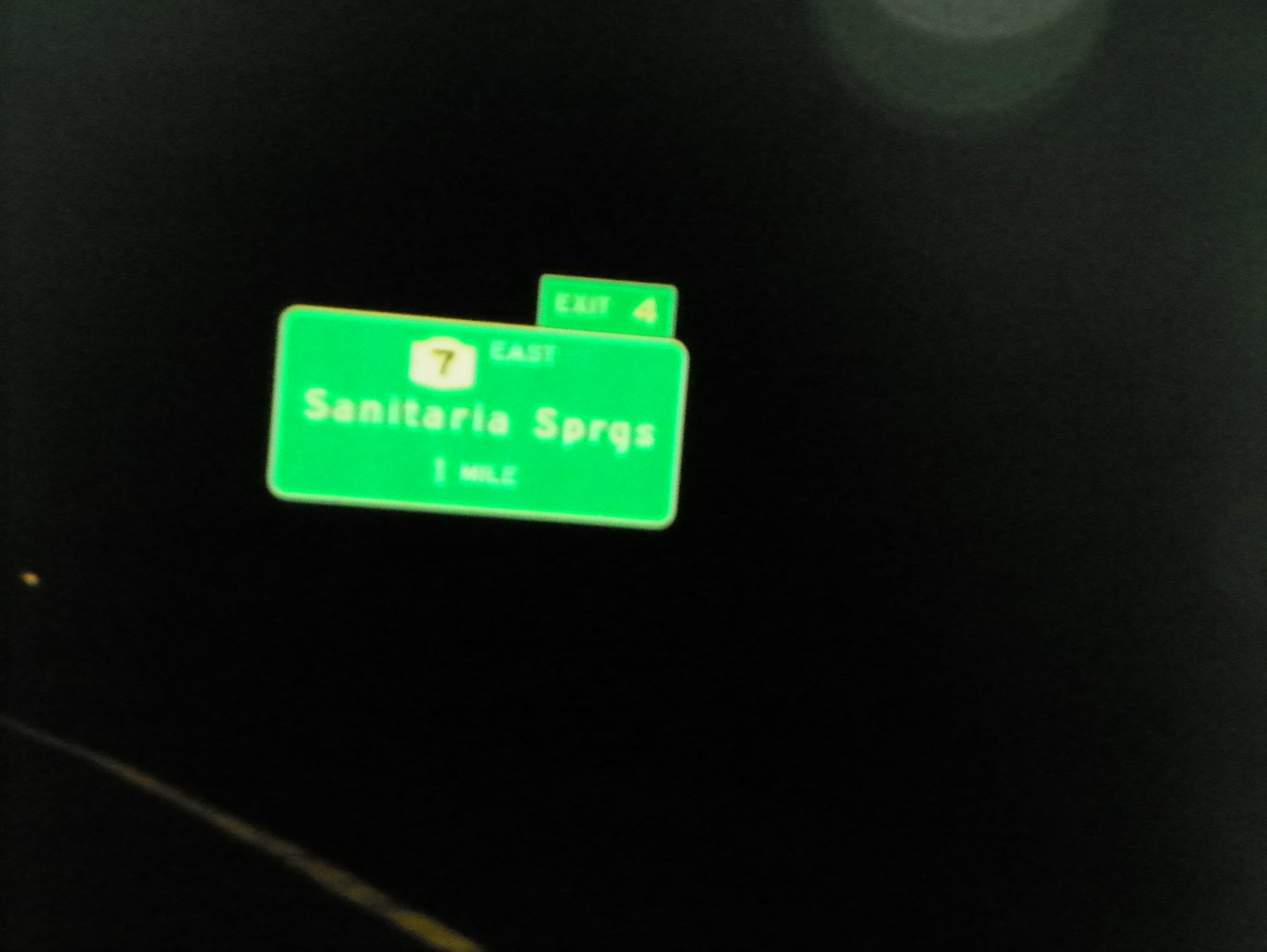The image depicts a nighttime scene with a predominantly black background, suggestive of the photo being taken outdoors, likely from a moving vehicle. The main focus is a green interstate road sign positioned slightly to the left and below the center of the frame. This sign indicates "Exit 4" for "Route 7 East" and reads "Santa Maria Springs," which is noted to be 1 mile away. In the upper right quadrant of the image, a source of light creates a circular halo effect, potentially moonlight. The lower left corner of the image features a partial view of the road, including a white edge line. Despite the blurriness indicating motion, the sign's details like its diagonal positioning and the text remain distinguishable.